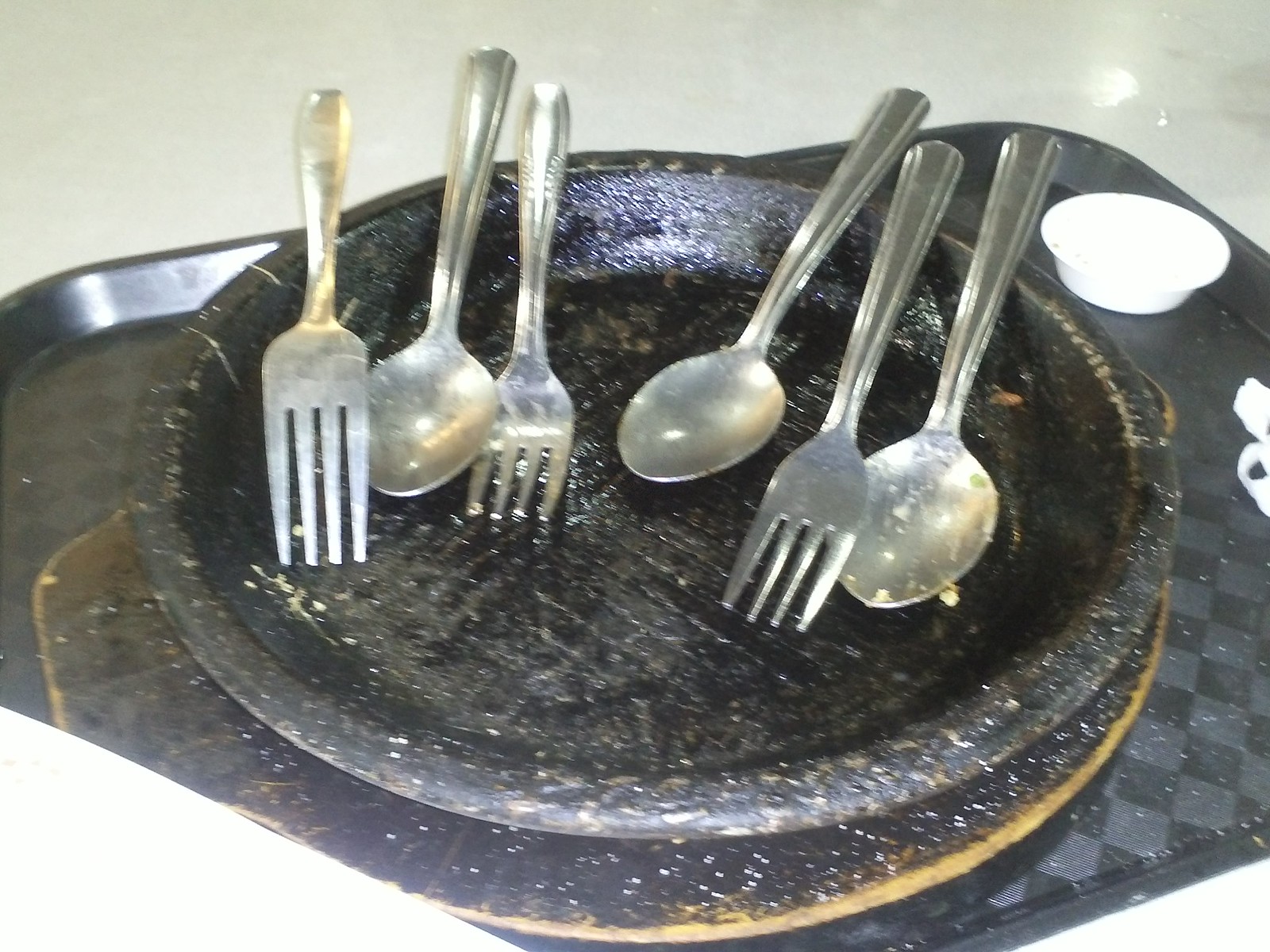The photograph captures a black tray with a distinctive black and gray checkerboard pattern. On the tray rests a black dish, above which sits another black bowl with gray dots printed on it. Positioned around the bowl from nine o'clock to three o'clock are six pieces of silver stainless steel utensils arranged in an alternating pattern of fork, spoon, fork, spoon, fork, and spoon. These utensils are not entirely clean, bearing remnants of a meal, possibly scrambled eggs. Situated on the outer edge of the tray is a small white plastic cup. The tray itself is placed on what appears to be a shiny white surface, reminiscent of the long tables used in schools.